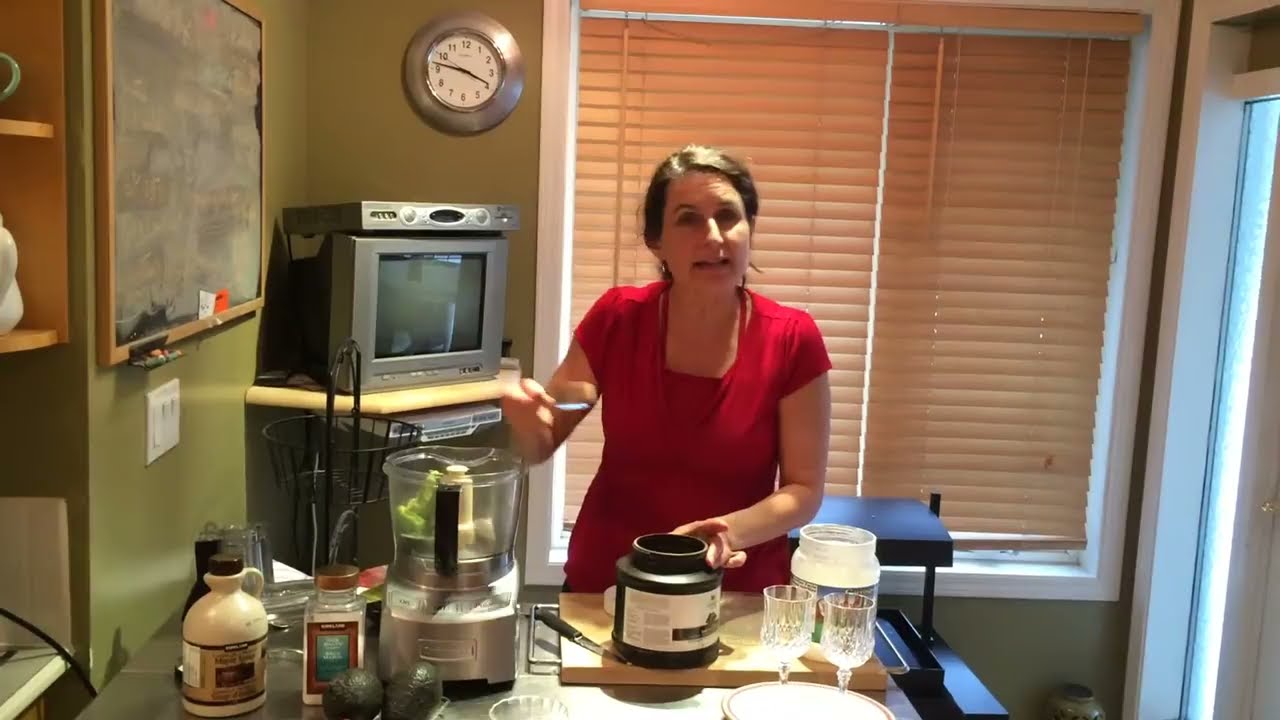In this detailed image, a young woman is standing in what appears to be a kitchen-like area, despite some ambiguity in its look. She is wearing a red short-sleeve blouse and faces the camera with her mouth partially open and her eyebrows raised, suggesting she's speaking, possibly during a video recording. Her right hand holds a spoon, poised over a black and white container with the lid off, indicating that she’s about to add its contents to a nearby silver blender. 

In the scene, there are two avocados in front of the blender, several containers, glasses, a plate, a glass bowl, a cutting board, and a knife—all tools suggesting she's making a culinary creation, likely a smoothie or shake. This workspace is part of a room with olive-colored walls, featuring a window with brown shades drawn closed. 

Behind her, there’s a white and silver clock on the wall, a chalkboard in the top left corner, and a small TV with a possible DVD player or VCR above it. To the right, an open doorway emits light, and nearby shelves add to the detail of this homey setting.